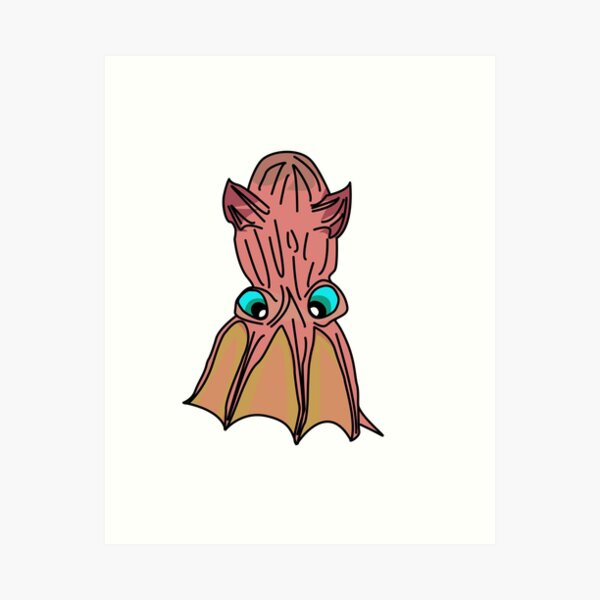The image features a hand-drawn, cartoonish creature that resembles a cross between an octopus and a bat, prominently centered within a plain white rectangle, which is itself set against a light gray background. The creature, about three inches high, is depicted with distinct red coloring and a brownish webbing between its appendages. Its eyes, strikingly blue with black pupils and white highlights, are centrally positioned on its body. Above these vivid eyes, the creature has a domed head with two pointy ear-like structures that could be interpreted as devil horns. Below its eyes, four webbed legs or fingers extend downward, intricately detailed with shades of mustard yellow and reddish pink. The overall appearance blends elements of a whimsical monster and a typical cartoon squid, presenting a unique and intriguing figure that stares directly ahead.